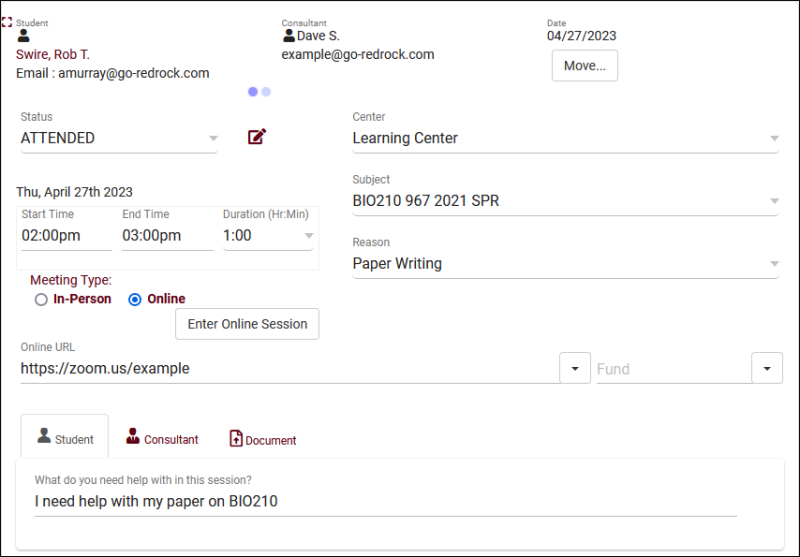A detailed screenshot from a computer screen displaying an online Zoom meeting interface, featuring key participant information and meeting details. In the upper left corner, the label "Student" appears in gray, accompanied by a simplistic human icon represented by a circle and curving lines for shoulders. Directly below, the name "Swire, Robert T" is prominently displayed in red, followed by an email address in black text, "email: A.Murray@go-redrock.com."

Across from Swire's information, the title "Consultant" is visible, next to another human icon, and the name "Dave S." with the email "example@go-redrock.com" listed beneath. To the far right, the field labeled "Date" shows "04-27-2023." Below this date, a button labeled "Move" is also visible. Further to the right, the "Status" section notes "ATTENDED" in bold, capitalized letters, adjacent to a red square containing a pencil icon. Detailed notes about the specific dates and times of the meeting appear below this icon.